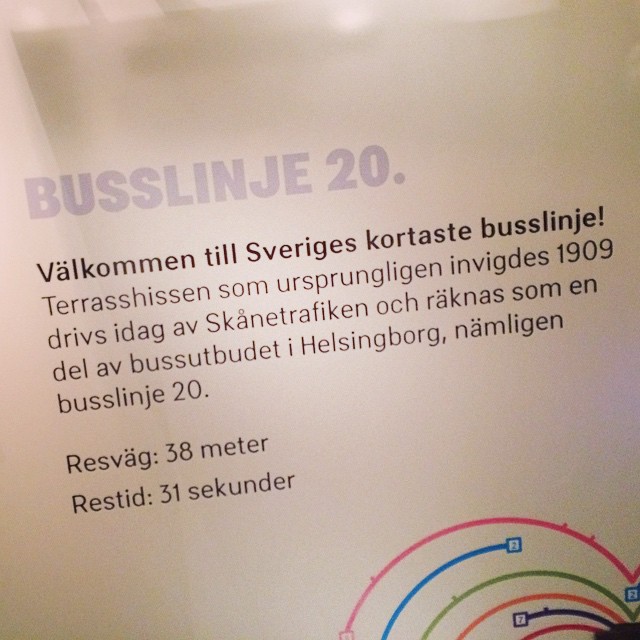The image is a close-up of a poster or flyer written in what appears to be a Germanic or Scandinavian language, possibly German or Swedish. The text includes both words and numbers, such as "20," "1909," "38 meters," and "31 Sekunder," which may refer to distance and time. The flyer seems to advertise a new bus line or route, suggesting improvements in travel speed and distance efficiency compared to previous routes. At the bottom right of the poster, there is a diagram featuring circular lines in different colors, each labeled with numbers, indicating various bus routes. The colorful diagram helps passengers distinguish between the different routes available.